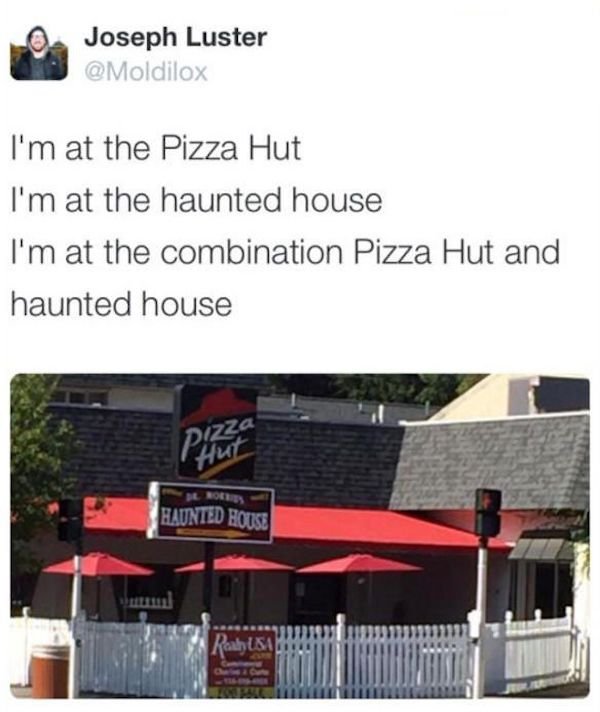This detailed caption describes a screenshot of a Twitter post:

The screenshot showcases a post by Joseph Lester (@MoldyLocks). The post features a humorous caption saying, "I'm at the Pizza Hut, I'm at the Haunted House, I'm at the combination Pizza Hut and Haunted House." Accompanying the text is a vibrant color photograph. The image depicts a distinctively unusual establishment—a combination of a Pizza Hut and a Haunted House. The building is adorned with a red awning and is surrounded by three red umbrellas and a white picket fence, which includes a red sign from Realty USA. The facade of the building prominently displays the classic Pizza Hut logo, while a rectangular sign below reads "Haunted House" in bold white letters. To the right of the image, an electronic crosswalk sign is visible, enhancing the urban outdoor setting. The varied color palette of the image includes gray, red, black, white, yellow, green, brown, and orange, contributing to the eclectic and whimsical atmosphere.